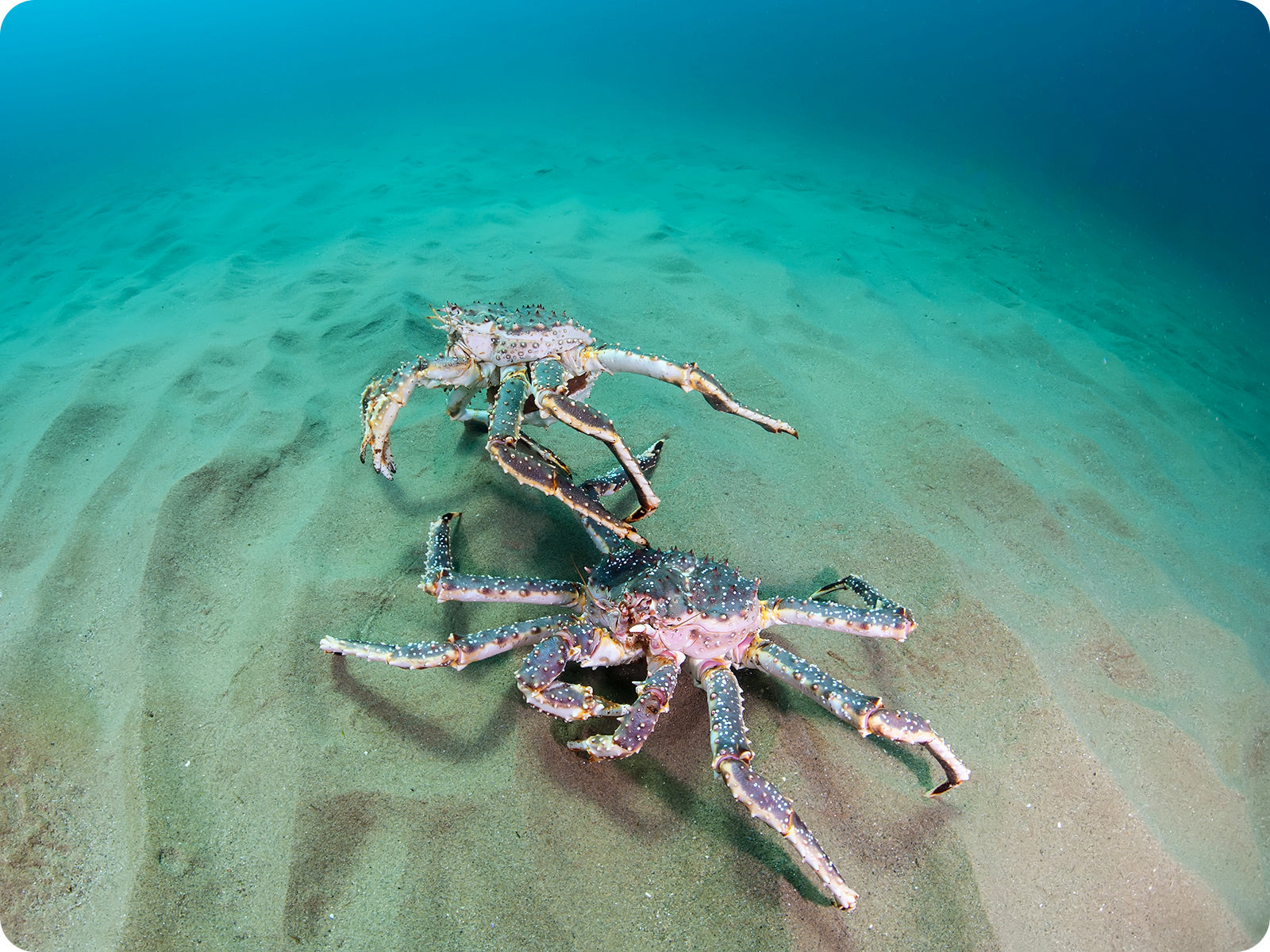In this captivating underwater scene, a rectangular photograph captures two starfish ensconced in a sandy bottom environment. The starfish in the foreground, a vibrant green with long, slender arms, commands attention as it stretches outward. Positioned slightly further back, another starfish is visible, displaying only four of its arms. The sandy substrate, featuring gentle wave patterns, provides a textured backdrop, suggesting it resides on the floor of an aquatic habitat. The upper portion of the image transitions from a dark blue at the top to a greener hue below, indicating the presence of water. The harmonious blend of colors and elements hints that the photo was likely captured with an underwater camera. The starfish appear poised, perhaps in anticipation or interaction, adding an element of intrigue to this underwater tableau.